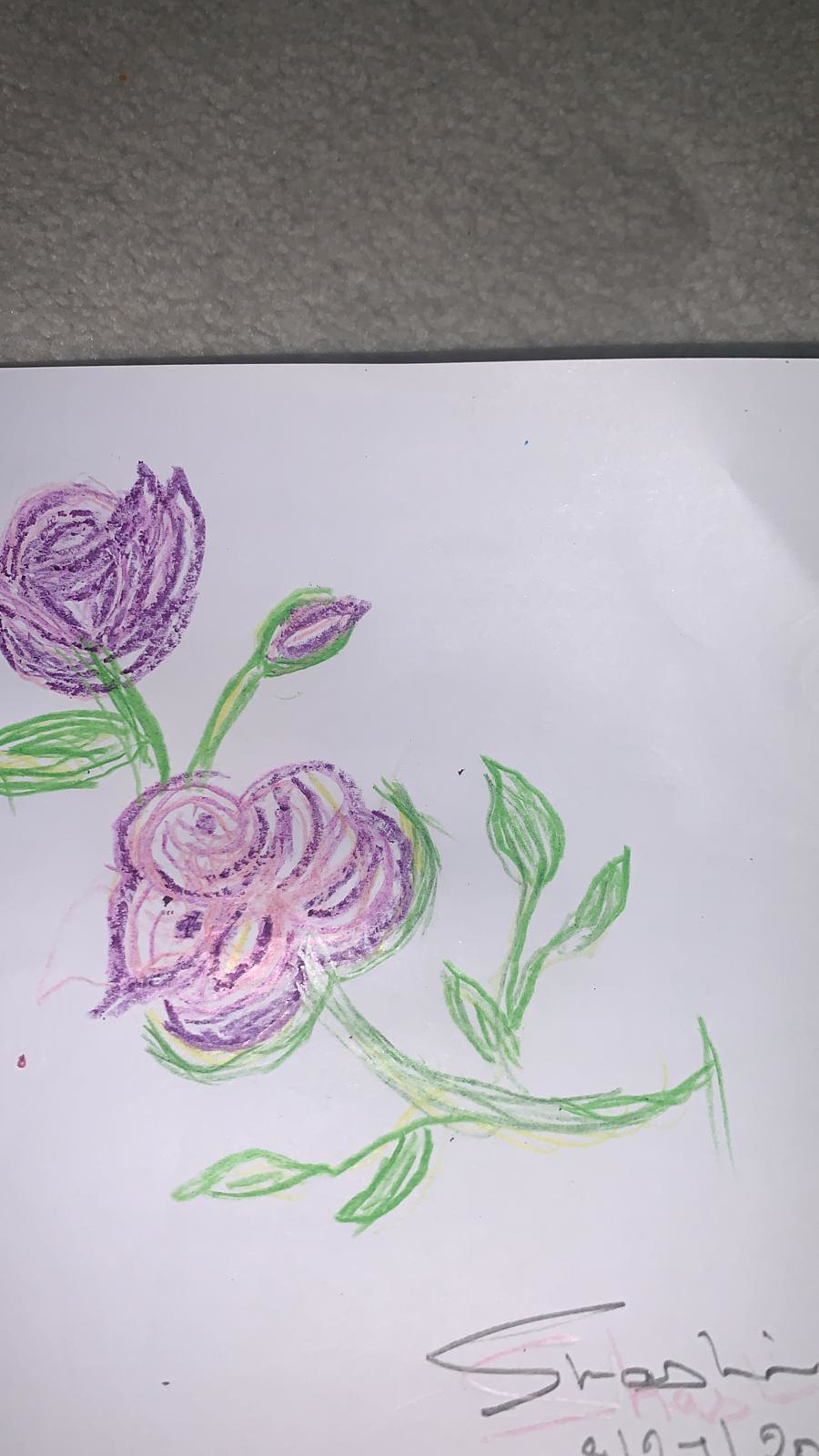This vertically-oriented photograph captures a crayon drawing placed on a white piece of paper, which itself rests on a grayish-tan carpet. The composition features two purple flowers, presumably drawn by a child, with evident crayon textures enhancing their whimsical appearance. The flowers, positioned towards the top-left and center-left of the drawing, are detailed yet childlike, with the upper flower resembling a tulip or bud and the lower flower fully bloomed with hints of pink and yellow. Both flowers sprout from green stems adorned with green leaves, some of which show yellow shading. The paper shows slight wrinkles at the top right corner, adding to its informal charm. The lower-right corner of the drawing includes a pencil signature, partially obscured and unreadable, along with traces of a date in pink crayon. The image is slightly zoomed in, cropping out parts of the left and right sides of the paper, yet retaining its delightful and innocent artistry.